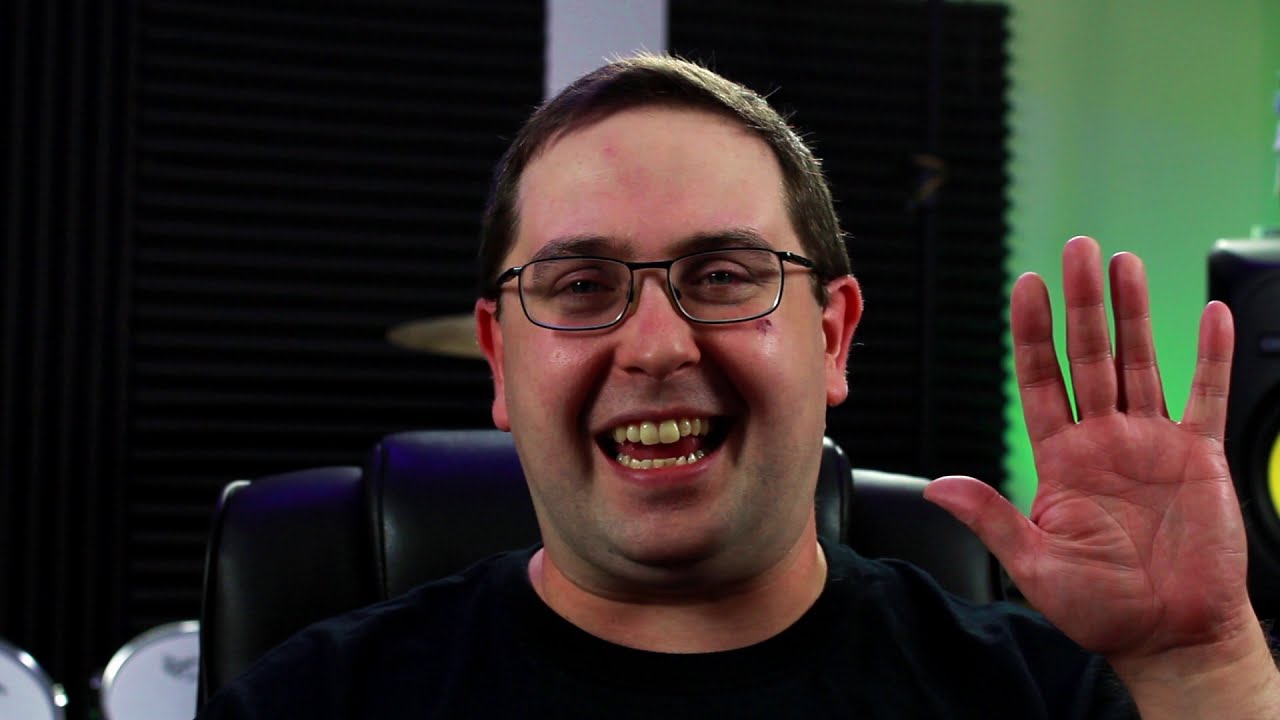This is an indoor photograph of a man seated in a comfortable, cushioned, dark indigo computer chair. The man, who is Caucasian with short brown hair and glasses, is smiling broadly with a cheerful expression, revealing his teeth. His left hand is raised in a friendly wave towards the camera. He is wearing a black t-shirt. Behind him, the wall features a unique design with a green light on the right side and a jagged-edged black panel in the middle. There are various objects around him, including items resembling parts of a drum set at the bottom left, suggesting that the setting might be a personal music studio. Overall, the image captures a joyous moment of the man likely intended for social media sharing.